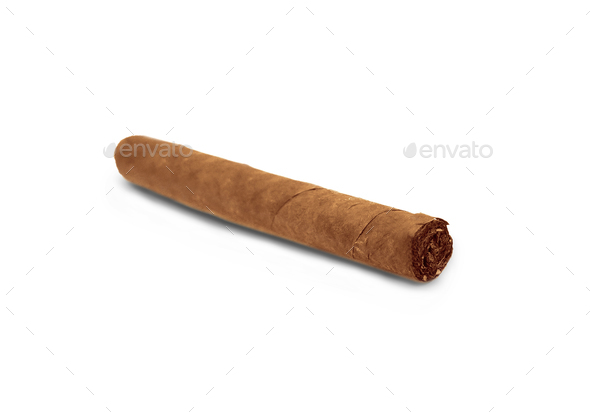The image features a singular brown cigar resting horizontally with a slight downward angle, prominently centered against a stark white background. The cigar appears hand-wrapped, showcasing its textured layers and varying shades of brown. The lighting end is nearest to the foreground, sharply in focus, while the rest of the cigar gradually blurs towards the back. Overlaying the picture is a faint, gray watermark with the text "Envato" repeated across the image in a dotted line pattern. No other objects or elements are present, emphasizing the solitary cigar and the Envato text watermark.